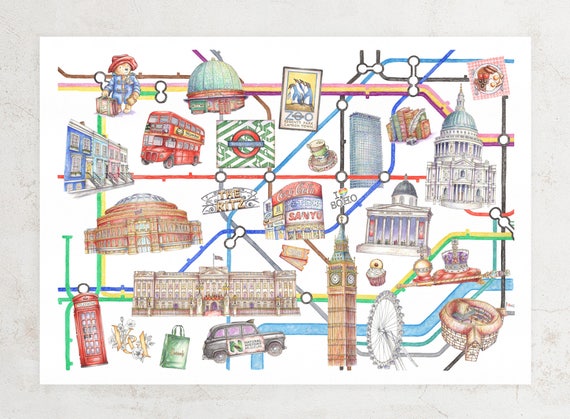This illustration, resembling a detailed map or game, features various elements related to London interconnected by vibrant, multi-colored lines. Displayed on a white paper with a light gray border, the image highlights landmarks and objects such as the red double-decker bus in the top left, the iconic red telephone booths at the bottom left, and the famous Big Ben clock tower. Buildings of different colors, including a depiction of the Capitol building and the London Eye, are scattered throughout the illustration. Additionally, there are food items, books, portraits, and other objects linked by lines in red, various shades of blue, black, purple, yellow, and pink. A key figure is a teddy bear in a blue attire holding a briefcase and wearing a red hat, positioned on the left side. The colorful lines mimic the appearance of subway lines in London, with the lines curving and varying in hue—peach, yellow, purple, blue, and dark blue—and small white circles marking specific points along them. The overall composition is both intricate and structured, offering a visually rich representation of different London-related themes and items.